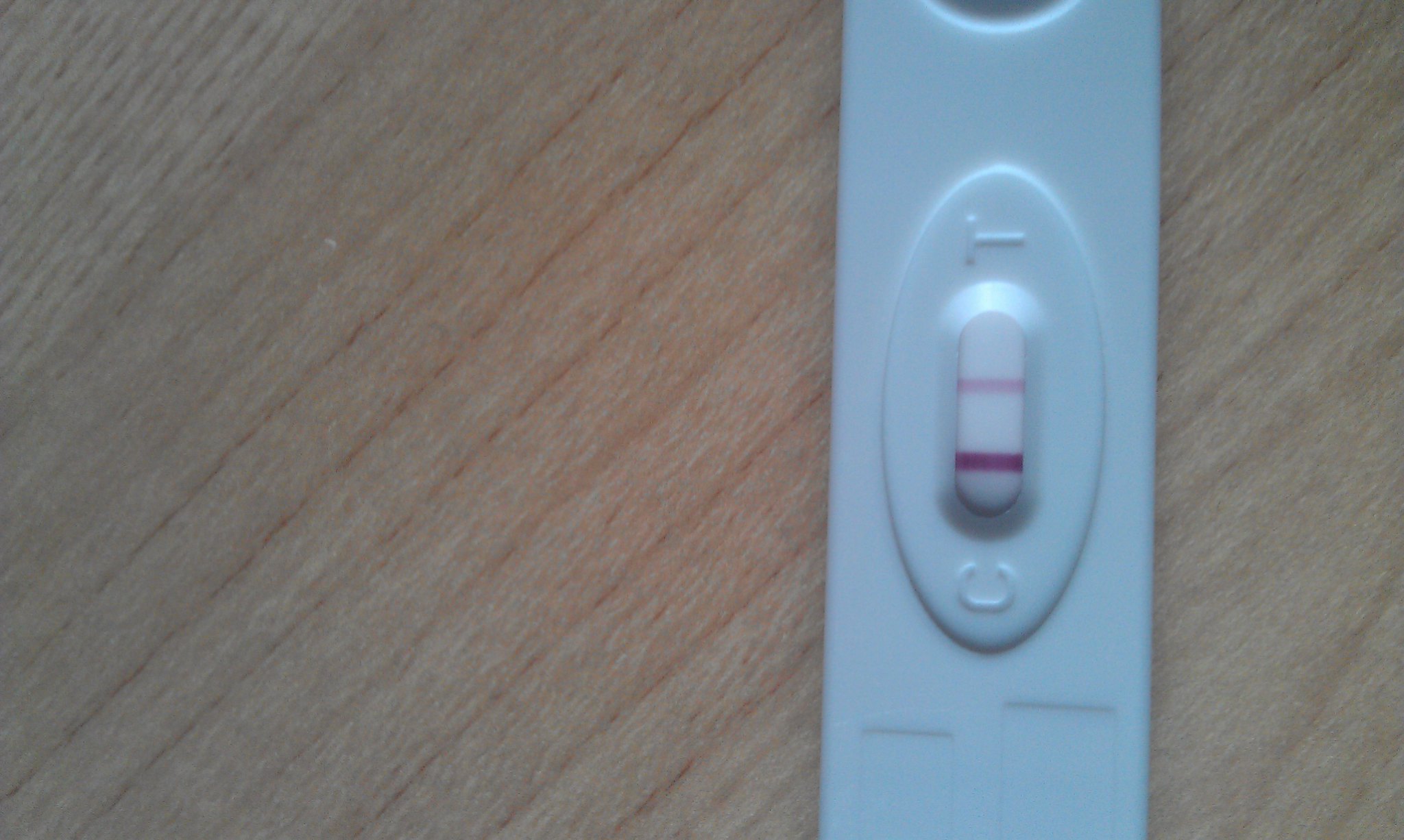The image showcases a white, rectangular object placed on a light brown wooden table that features visible grain lines. The table's natural wooden texture contrasts with the sleek, white surface of the object. This object has an upper segment labeled with a 'T' and a lower segment marked with a 'C.' Notably, there is an oval indentation situated between these segments. Running horizontally through the middle of the object are two distinct red stripes: the upper stripe is a dark red, while the lower one is light red. The composition of the object, displayed against the wooden backdrop, highlights its clean lines and the pronounced red detailing.